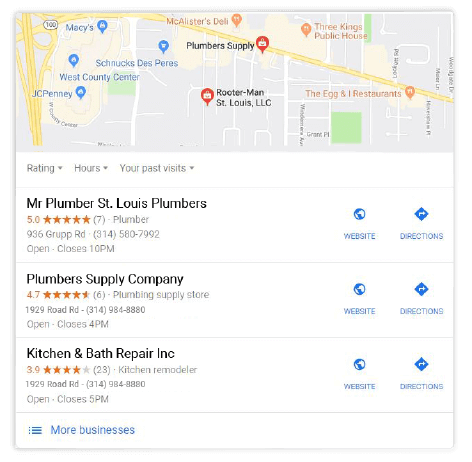**Detailed Descriptive Caption:**

The image depicts a Google search results page focused on plumbing-related businesses. At the top of the search results, there's a map displaying several location pins. Key highlighted locations include Macalester's Deli, Three Kings Public House, Eggs and Restaurant, and several plumber-related establishments. Notable pins are for St. Louis Plumber Supply, assigned with a 4.7-star rating based on six reviews, and identified as a plumbing supply store that closes at 4 PM. Also listed, but not visible on the map, are Mr. Plumber, a plumber with a 5-star rating from seven reviews who operates until 10 PM, and Kitchen and Bath Repair Inc, a kitchen remodeling service with a 3.9-star rating from 23 reviews. The text also mentions other landmarks like Rochester, Maine, and West County Centre, with subtle annotations indicating their relation to Macy's store and similar establishments. The image’s primary focus remains on providing detailed business information, such as addresses, contact numbers, operational hours, and direct links to websites and directions.